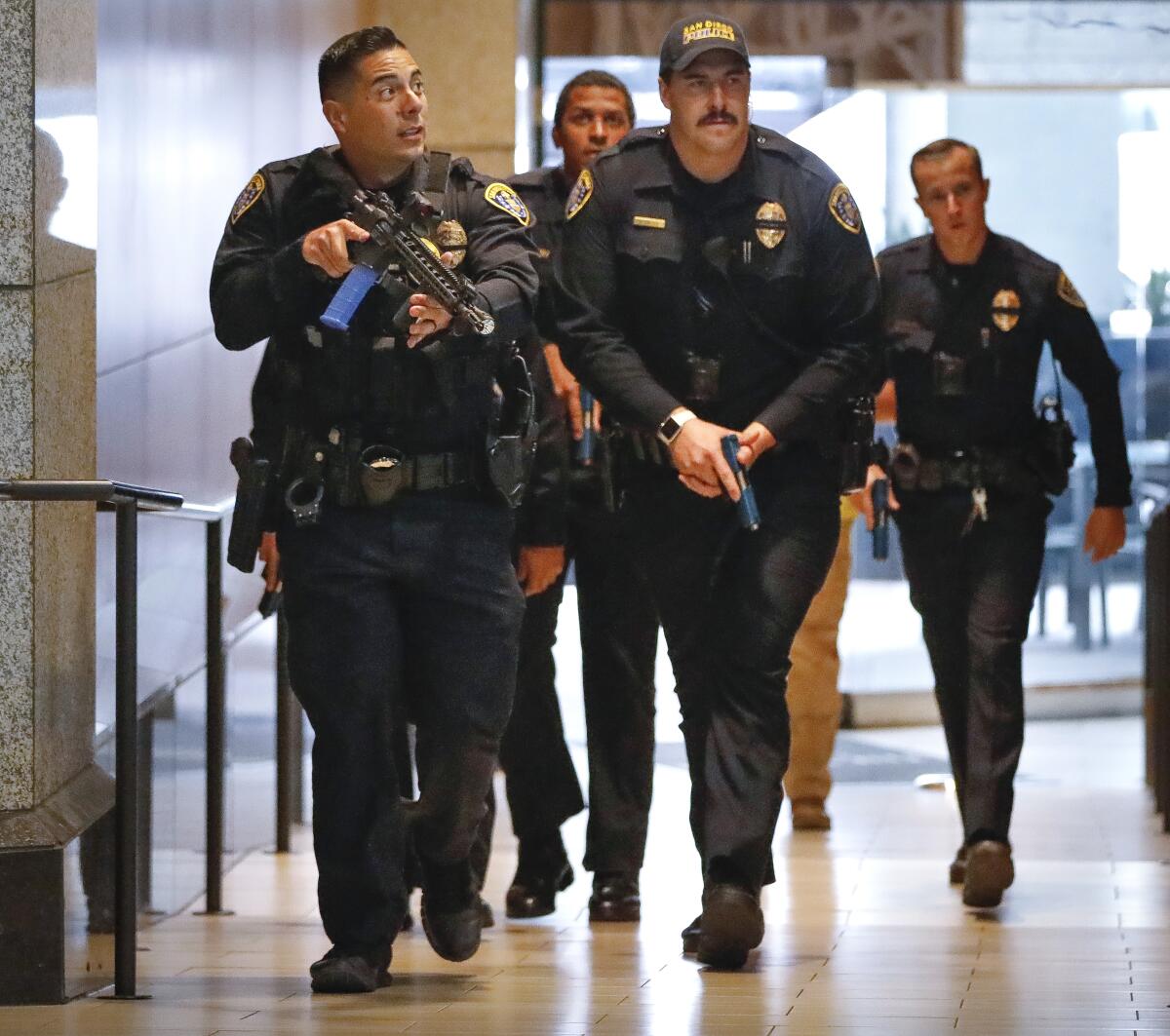The image features four police officers, dressed in navy blue uniforms and dark shoes, walking purposefully through a sunlit hallway with a reflective tan-colored linoleum or tiled floor. Each officer has their weapon drawn; three brandish blue-handled pistols while the man on the front left, with short black hair, carries a more substantial assault weapon alongside a holstered gun and orange-detailed handcuffs on his belt. To his right, a white officer wearing a navy baseball cap with an orange or yellow inscription grips a blue handgun, and his mustachioed expression is intensely focused. Behind them, one officer, partially seen, is of African descent with short black hair, and the other, with short brown hair, is also holding blue pistols. An additional fifth individual, only discernible by their brown pants and shoe, trails them. The path they walk along is next to a black metal railing beside marble or limestone-colored pillars, their serious expressions and aggressive posture suggesting they are responding to an immediate threat. Sunlight filters through large windows, casting reflections and highlighting the tension in this captured moment.